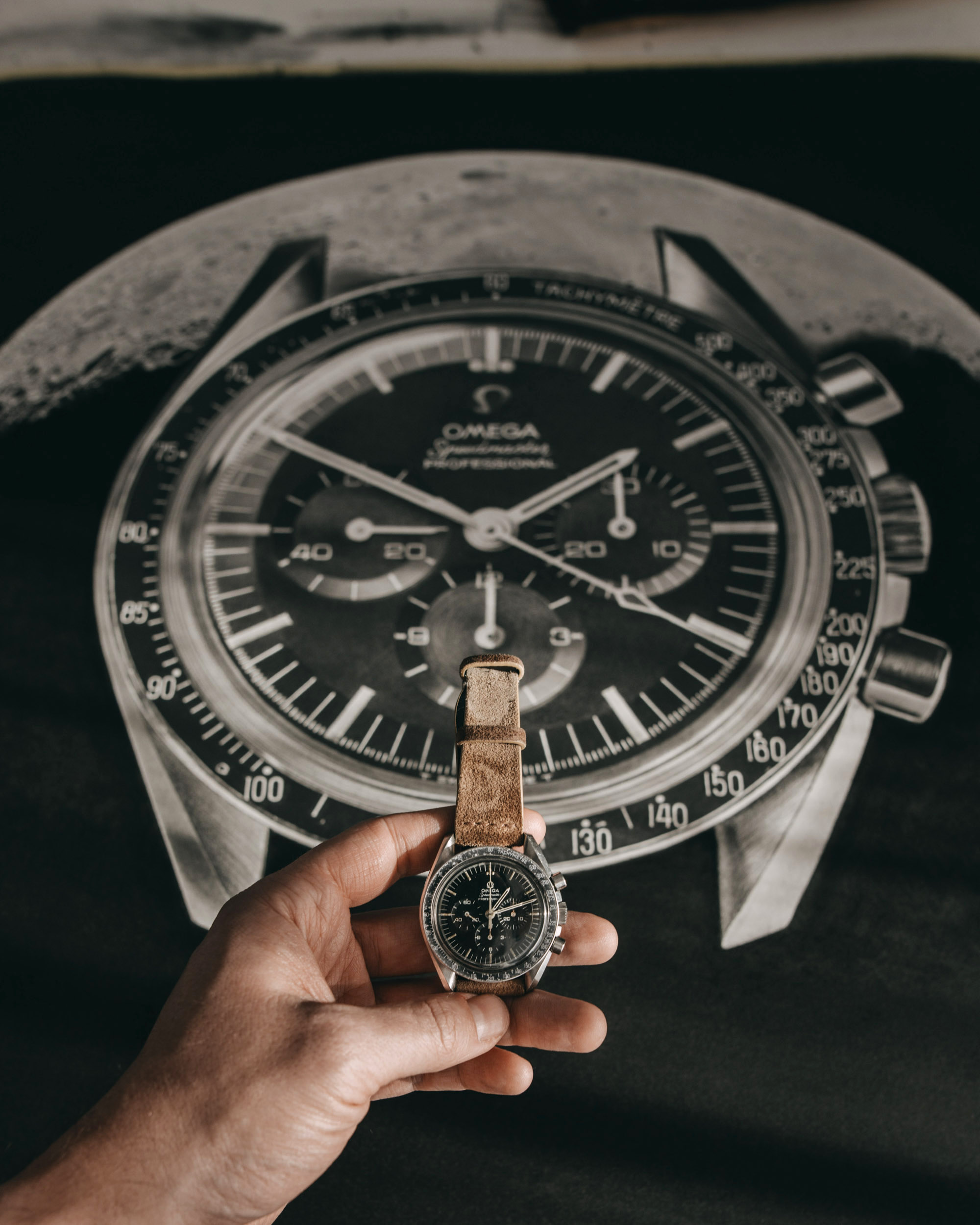In this detailed photograph, we see a close-up of a person's left hand emerging from the bottom left corner, holding an old Omega watch. The watch features a worn, brown leather strap and a silver stainless steel case. Its vintage design is accentuated by traditional, non-digital hands and winding knobs on the right side. The face of the watch is black with additional sub-dials, and it displays the time as 1:50 (or 10 minutes to 2 o'clock). The name "Omega" is prominently inscribed on the dial, along with some other, less clear inscriptions.

In the background, there is a large, zoomed-in image of the same watch, providing a detailed view of its black face and Omega branding. This oversized depiction includes a partial moon image, suggesting a possible "moon landing" or "space edition" theme. The background is predominantly dark, enhancing the visibility of the moon's detail at the top.